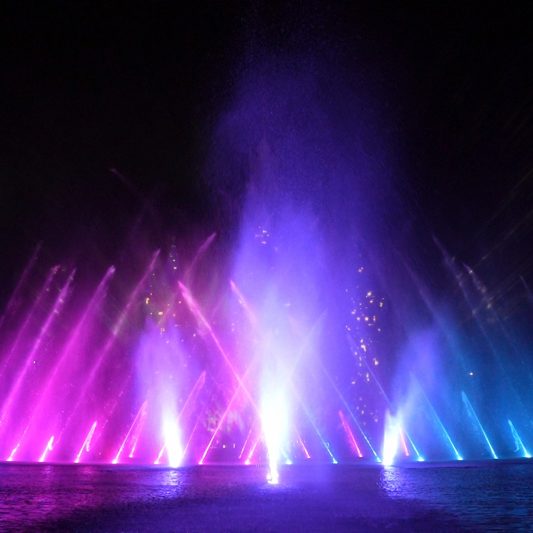This vibrant, square photograph captures a mesmerizing nighttime light show, set against a pitch-black sky. The composition centers around a body of water that runs horizontally along the bottom edge of the image, reflecting the dazzling display above. Three intense white beams of light shoot straight up from the water, creating a striking vertical presence. To the left, magenta and hot pink streaks of light ascend towards the center, adding a burst of vivid color. On the right, brilliant blue lights rise diagonally across the image, intersecting with the other beams and adding dynamic movement. Hovering above the lights is a mist suffused with a captivating blend of bluish and purplish hues, enriching the scene with an ethereal glow. The overall effect is a breathtaking spectacle, likely from a celebratory event or special occasion.